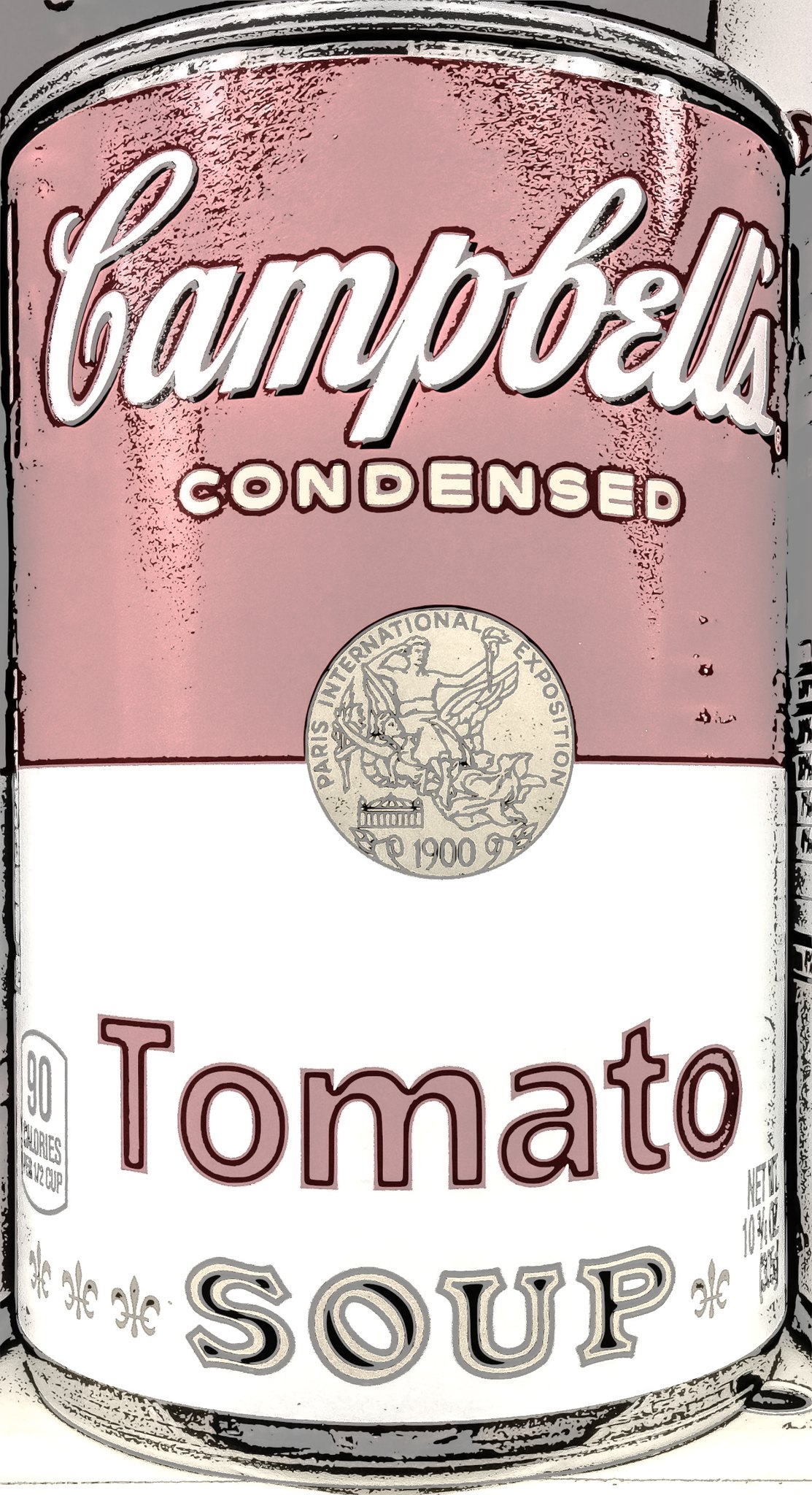The image showcases a digitally altered, close-up view of a Campbell's Tomato Soup can. The can is presented straight-on, featuring a standard red and white label that appears severely washed out, giving the red a nearly pink hue. The Campbell's brand name is prominently displayed at the top in a large, white, cursive font, followed by the word "condensed" beneath it in smaller, golden capital letters. Central to the label is a gold seal with the inscription "Paris International Exposition, 1900," which has also been affected by the wash-out, appearing yellowish and flat. Below the seal is the word "tomato" in bold red letters on a white background, and under that, the word "soup" in black. The lower portion of the can includes nutritional information, stating "90 calories per serving." The image has a grainy, overexposed, and highly reflective appearance, likely due to digital manipulation, possibly through a posterized or high-contrast filter. The photo is cropped closely around the can, with faint indications of adjacent cans on either side, blurring into the periphery.